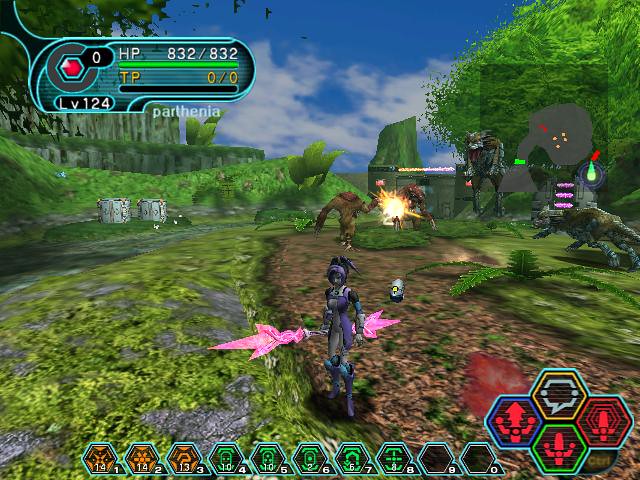Screenshot from a computer game featuring the central player character clad in intricate purple gear. The character wields a distinctive pink stylized weapon in their right hand. The screen is bustling with numerous maps and HUD elements, providing a wealth of in-game information. In the lush, green background with a clear blue sky, two large brown beasts are seen battling each other, adding dynamic action to the scene. The HUD in the top left corner displays the location name "Parthenia."